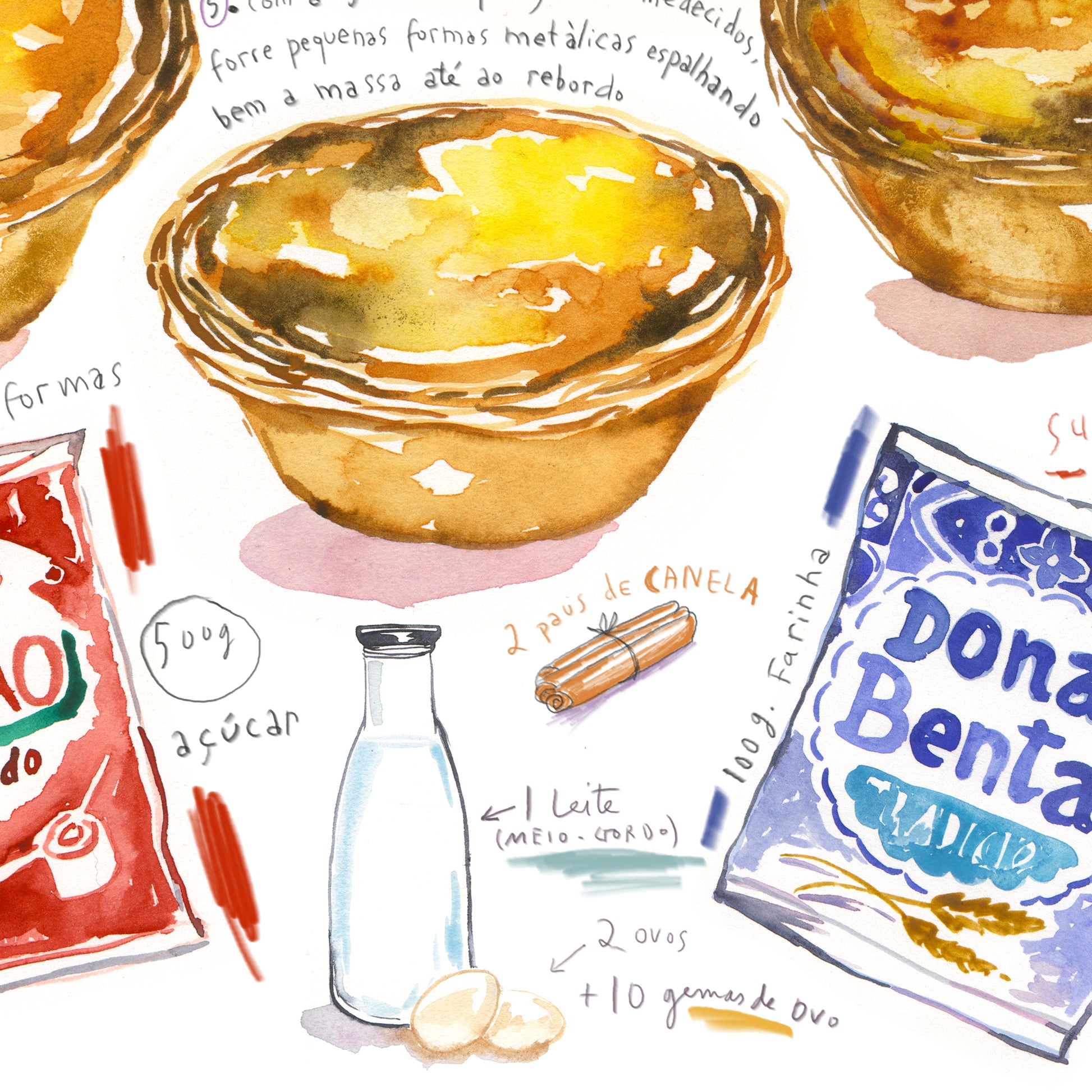The image features a beautifully detailed watercolor illustration of a recipe, primarily written in Portuguese. The central focus is on the ingredients and instructions for making a custard-like dish, possibly flan or hand pies. The artwork includes a sketch of round pie crusts that resemble small cups filled or topped with custard. Accompanying the drawing are various ingredient illustrations and notes: a milk jug, two eggs (labeled "ovos"), three pieces of tied cinnamon sticks ("paus de canela"), and a blue flour bag marked "100 G Farinha" with the brand "Dona Benta." There's also a small graphic of a bag indicating "4 months" and "500 grams de açúcar" (sugar). Pencil markings at the top include a circled number five and other handwritten details. The combination of charming watercolor visuals and pencil annotations creates a unique, half-drawing, half-writing instructional piece.